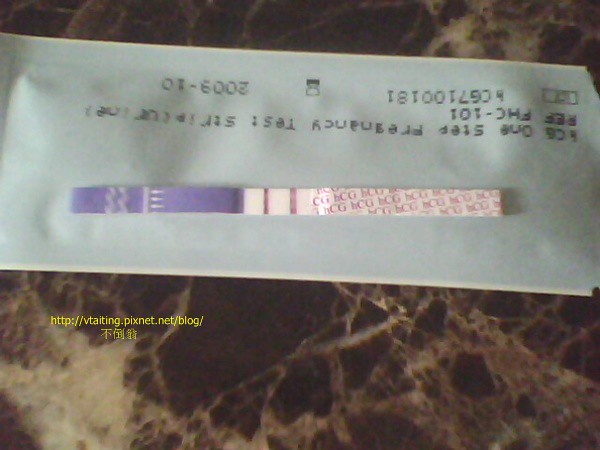This image features an upside-down label displayed against a hard surface with a scattered, black and gray design, suggesting it might be a table or counter. The label itself is light blue and prominently features a long rectangular strip. The left side of the strip is blue and adorned with small white arrows pointing left. Transitioning to the right, the strip morphs into a label with the bold red font "HCG." Central to the label are two vertical red lines. Below the main strip, a website URL, "vtiting.pixnet.net," is clearly visible in yellow font. Additionally, the label is marked with a date in the corner, which reads "2009-10."